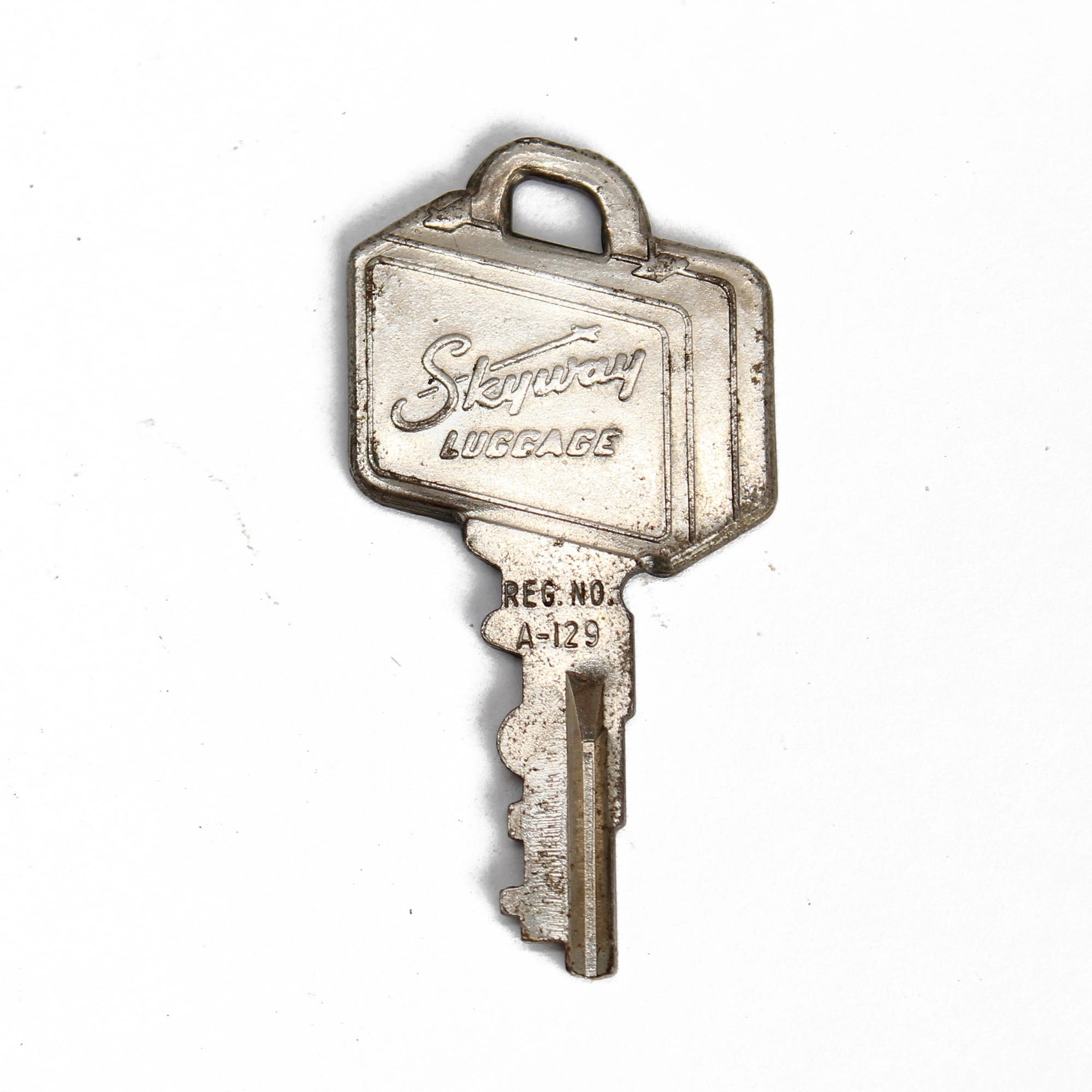The image depicts an antique key that has clearly seen better days, exhibiting a textured surface with speckles of gray, black, and rust. The most striking feature of the key is its unique head, crafted to resemble a piece of luggage, complete with a small handle where the keychain hole is situated. This rectangular luggage design is elaborately engraved with the words "Skyway Luggage," featuring a stylish shooting star crossing through the "S" and the "K" of "Skyway." Below this intricate design, the shank of the key is marked with "REG. NO." and the code "A-129." Despite its worn and pitted appearance, characterized by silver-gray hues interspersed with darker patches, the key remains a fascinating example of detailed craftsmanship and functionality.